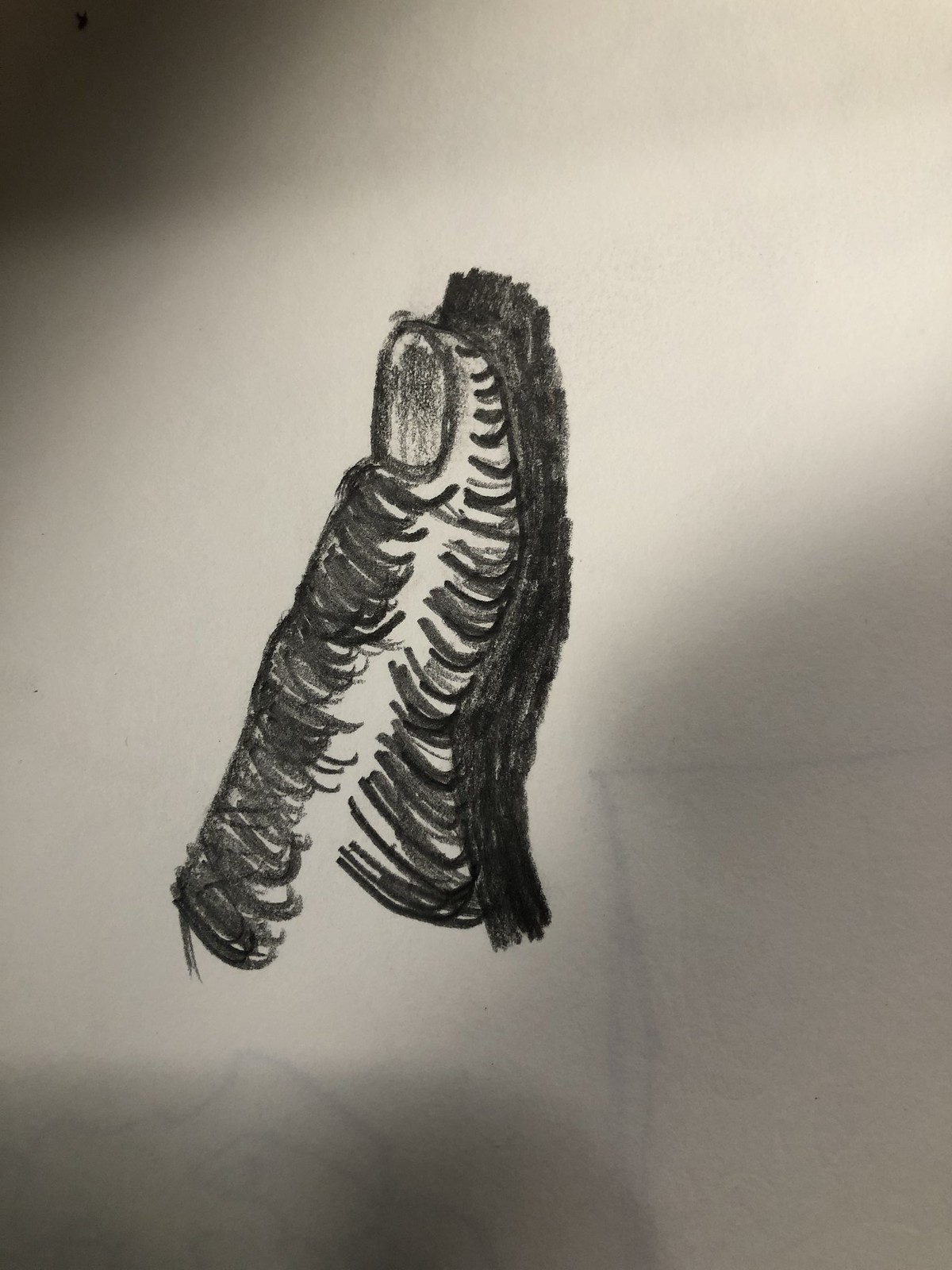This close-up image captures a vibrant crayon sketch depicting an intense scene of two caterpillars in what appears to be a fight. The left caterpillar features a distinctive, round head shaded in dark tones, giving it a dynamic and emotive appearance. In contrast, the right caterpillar resembles a typical caterpillar with numerous legs meticulously drawn, emphasizing its segmented body. The sketch is framed within a partial view of the paper, suggesting a zoomed perspective that focuses on the caterpillar confrontation. The right side of the image reveals a faint trace of another drawing—a rectangular shape bleeding through the paper—hinting at an underlying layer of creativity. Additionally, the top left corner of the image is shrouded in a large shadow, adding depth and a sense of mystery to the artwork.